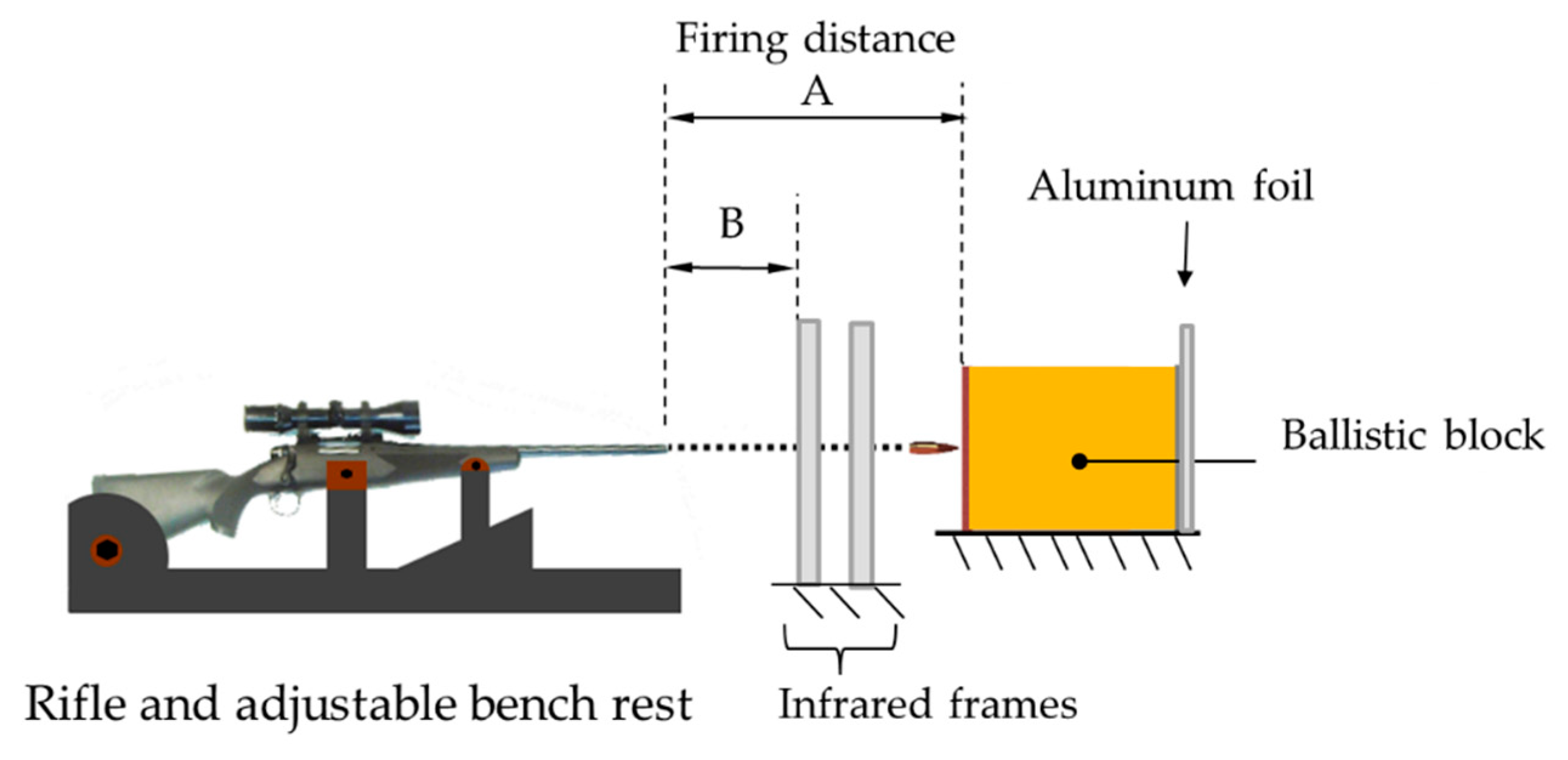The horizontal rectangular image shows a detailed setup of a rifle mounted on an adjustable bench rest. The rifle is primarily gray with some red markings on its side and features a telescopic sight on top. In front of the rifle, there's a ballistic block, followed by a piece of aluminum foil. Between these two elements, the term "infrared frames" is indicated. Above the entire setup, there are labels and arrows showing the firing distances, marked as A and B, respectively. Additionally, the diagram displays detailed instructions on how to aim and fire the rifle, with dotted lines extending from the tip of the rifle through the infrared frames to the ballistic block. Yellow blocks and other annotations are also present to depict various components and measurements involved in the firing process.